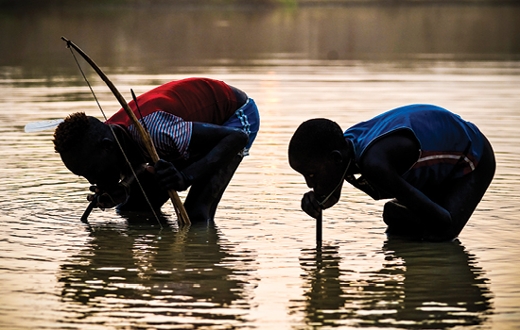This photo depicts two black males standing knee-deep in a calm body of water, likely a pond or lake, with gentle ripples reflecting the daytime sunlight. They are both bent over, seemingly drinking from the water using long, reed-like straws. The man on the left, dressed in a blue shirt and shorts, is holding a bow and arrow while using the straw. He has short hair. The man on the right, clad in a red shirt with stripes and shorts, has frizzled, spiky hair and is focused on the straw in the water. The sun glimmers on the water's surface, contributing to a tranquil ambiance. The bright, summery clothing and natural setting suggest a warm day, possibly in a rural or secluded area, potentially in Africa.